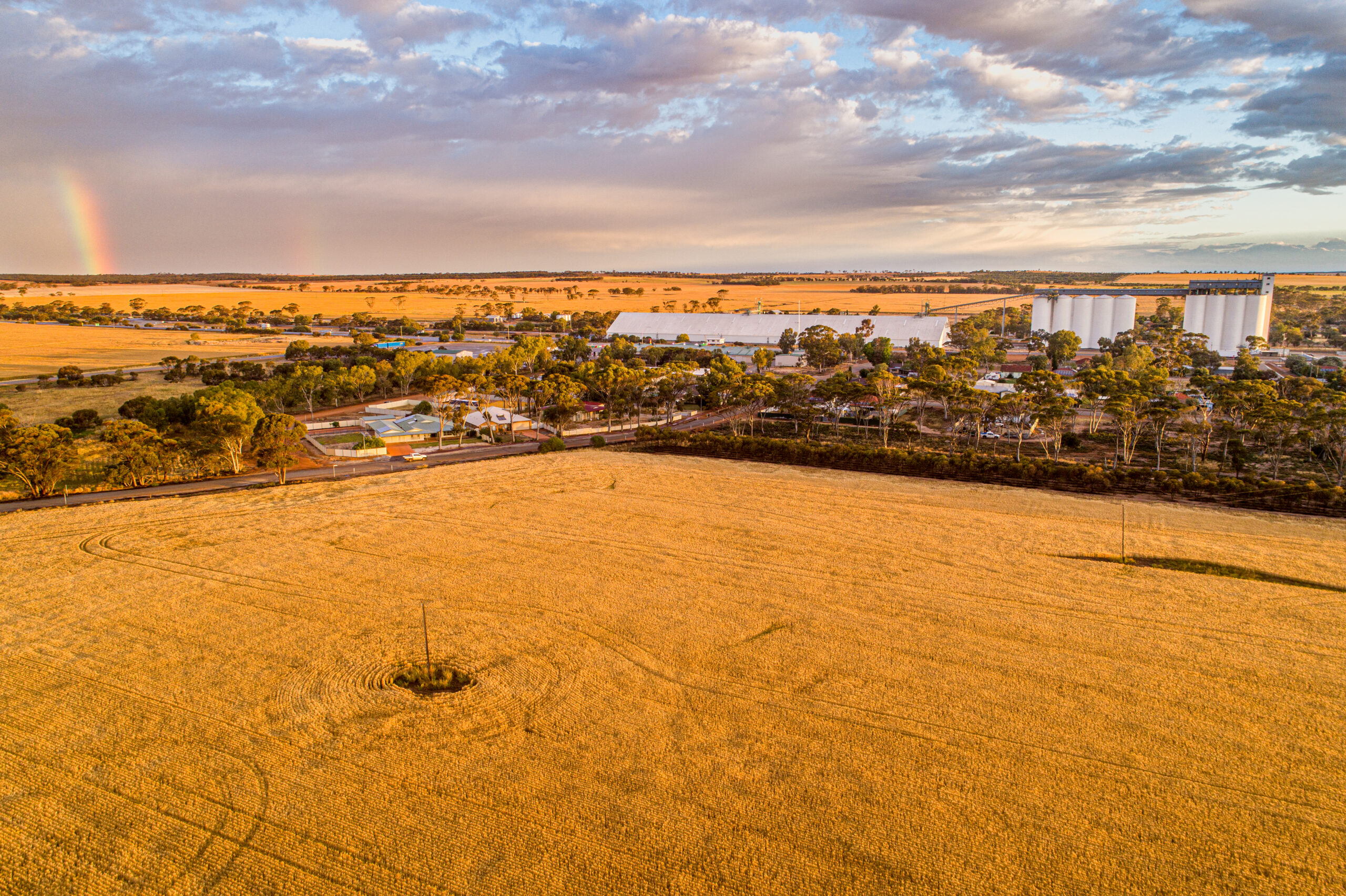The image showcases a farm landscape with a recently harvested agricultural field dominating the foreground. The field, which displays a rich ochre yellow color with numerous trails and tracks from harvesting vehicles, extends up to the central part of the image. Near the left-hand side of the field lies a small, circular green and black object. Surrounding the field are vibrant green trees, and to the left, a gray parking lot bordered by light brown edges can be seen. In the far distance, other golden fields and patches of trees are visible. The farm's infrastructure, including several white buildings, silos, trees, and fences delineating different sections of the property, is situated in the background. The sky above is mostly filled with gray clouds that part to reveal patches of blue, and in the upper left-hand corner, a rainbow arcs gracefully from the sky down to the ground.